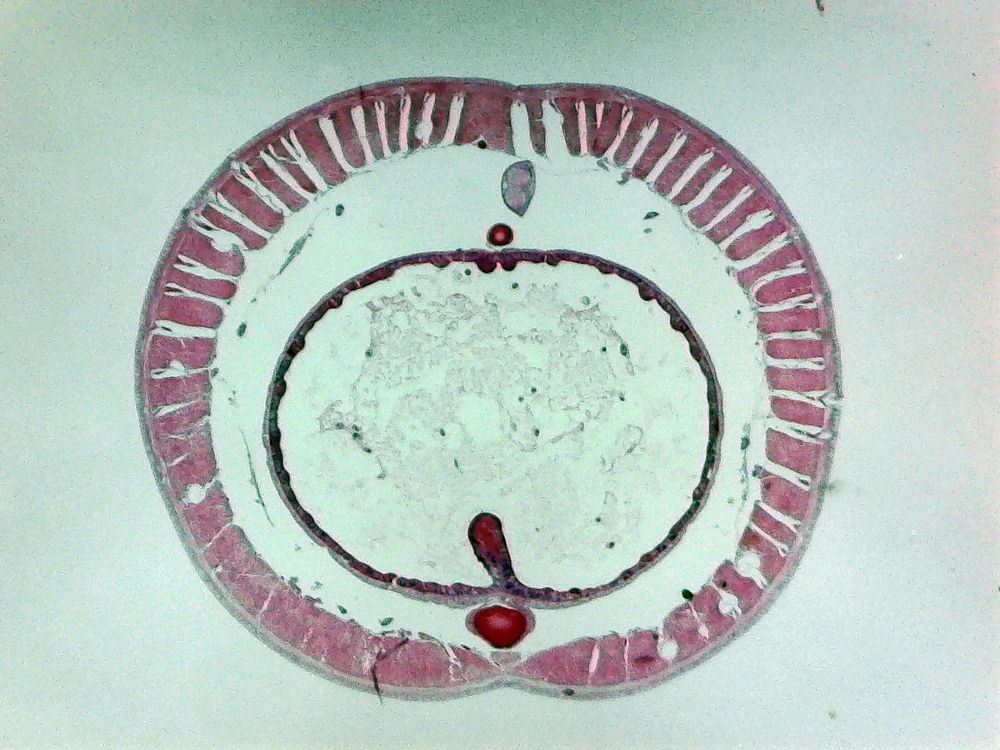In the image, there's a central focus on an abstract, almost apple-shaped figure on a predominantly white canvas with varying shades of green hues created by ambient lighting. The central circle, reminiscent of a not completely round plate or a cell, features an intricate border design with thick waves in a dark red to gray gradient. This outer border transitions into an inner stripe pattern which extends sporadically toward the center in red and white streaks. The inner circle showcases a ragged, worn texture with visible signs of wear and tear. At the top of this inner circle, a small green dot and a couple of red dots are distinctly visible. Toward the bottom of the inner circle is another smaller outline in burgundy and dark brown, enclosing additional splatters of green paint resembling a whipped dessert with tiny green specks. The entire composition is set against a light greenish-gray background, enhancing the abstract and somewhat cellular appearance of the artwork.